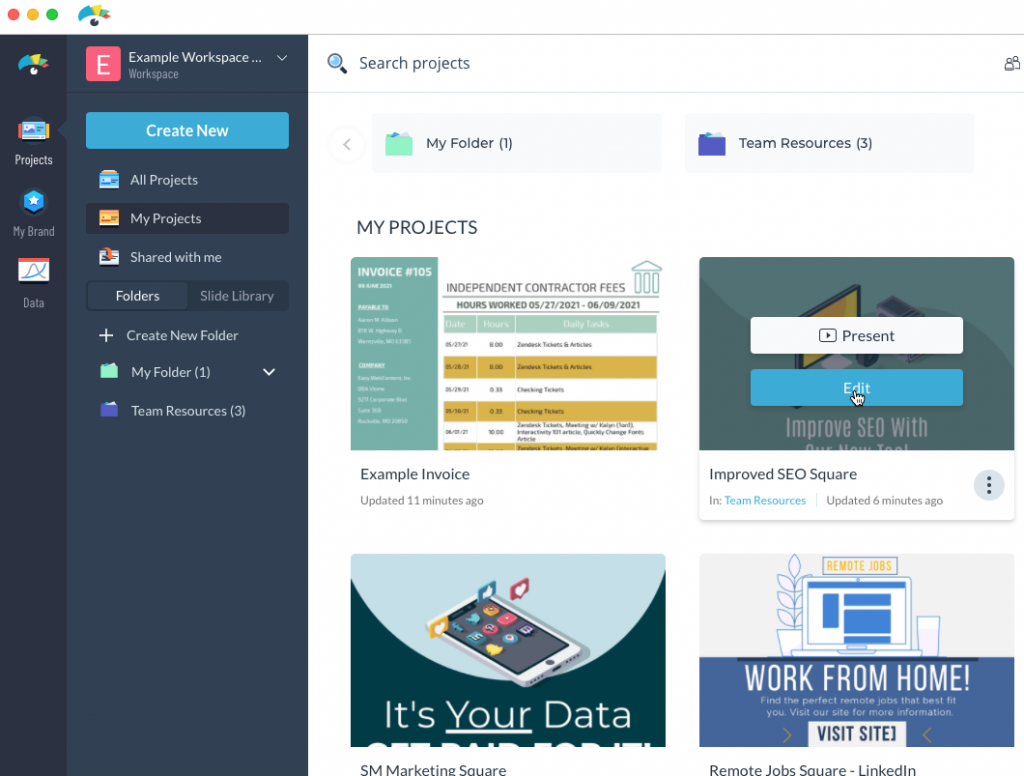This screenshot depicts a website's user interface with a complex and detailed layout. In the upper left-hand corner, there are three dots (red, yellow, and green) commonly used for window controls. Next to these, there is an unknown logo comprised of blue, yellow, green, and red pieces arranged in a manner resembling an eyebrow over an eye.

The main section is divided into three distinct columns. 

**First Column (far-left):**

- The background is black.
- The same logo appears at the top.
- Below the logo, there are three options listed vertically: 

  1. Projects (with an arrow indicating a submenu)
  2. My Brand
  3. Data

**Second Column (middle):**

- The background is a shaded light black.
- At the top, it reads "Example Workspace" with a down arrow next to it.
- A prominent blue button labeled "Create New" in white text is prominently displayed.
- Below the button:
  - "All Projects"
  - "My Projects" (highlighted in black, indicating it is currently selected)
  - "Shared With Me"
- Further down, there are two buttons labeled "Folders" and "Slide Library".
- Under the "Folders" section, options provided are:
  - "Create New Folder"
  - "My Folder 1"
  - "Team Resources 3"

**Third Column (far-right):**

- This column is a detailed project list linked to the selected "My Projects".
- At the top, a search field titled "Search Projects".
- Listed items include:
  - "My Project"
  - "Invoice 105, Independent Contractor Fees"
  - On the right side: "Improved SEO Squared"
  - Below that: "SM Marketing Square"
  - On the right side: "Remote Job Square, LinkedIn"

This clean, organized user interface enables efficient project management and accessibility to various user and team resources.